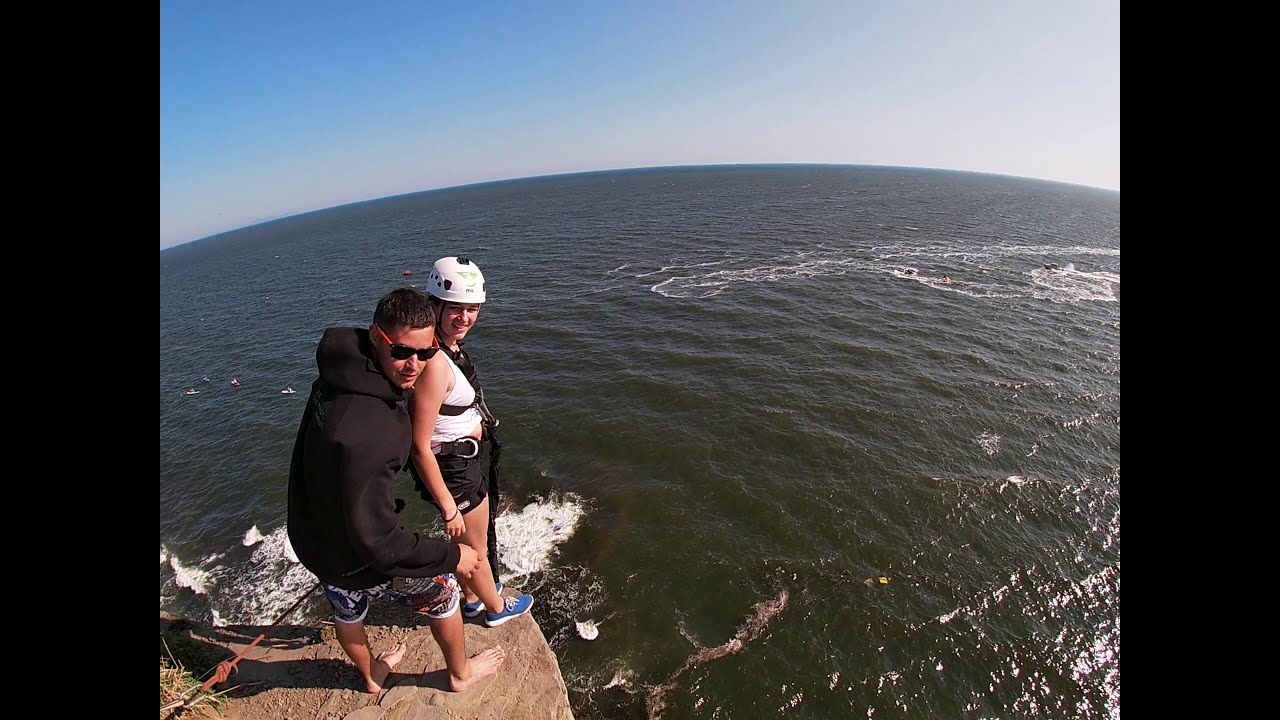The image depicts a sunny, clear day with a vast expanse of murky, brownish water extending into the horizon, beneath a vivid blue sky. Situated at the lower left corner of the photo, a woman stands at the edge of a tall cliff, appearing ready for a bungee jump. She is equipped with a white helmet, a white tank top, black shorts, and blue sneakers, securely strapped into a protective harness with a rope attached to her. Smiling, she looks back towards the camera. Behind her, a man who could be her instructor is standing barefoot on the cliff. He is wearing a black hoodie, shorts, and sunglasses, with short brown hair. Both of them are looking back at the camera, capturing a moment of anticipation and excitement. The wide lens of the photo adds a rounded, almost oval effect to the image, emphasizing the curvature of the horizon and the expansive body of water below.